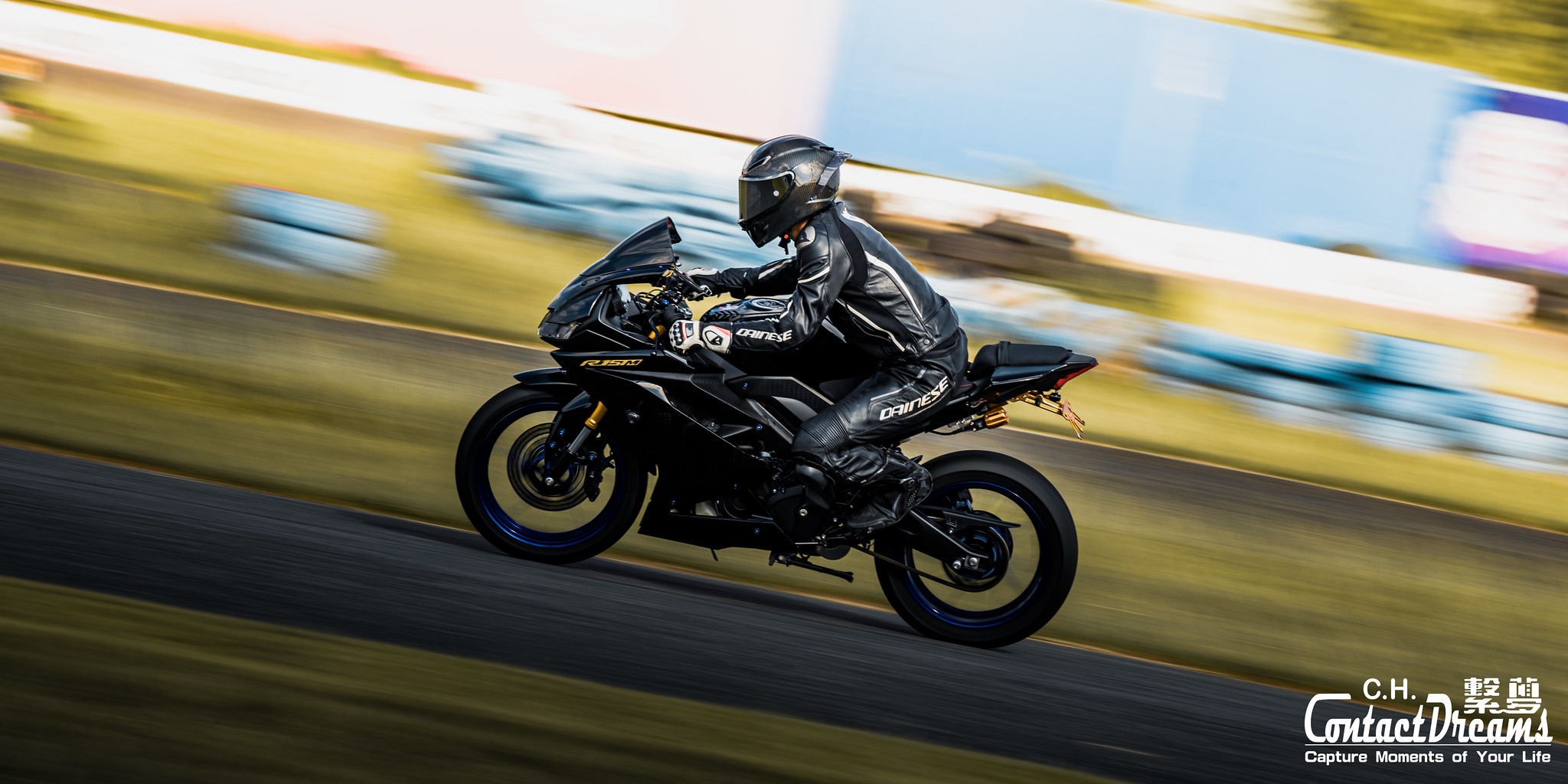This dynamic and visually striking photograph showcases a motorcyclist on a sleek, black sports motorcycle, evocative of an advertisement. The motorcyclist, whose gender is indistinguishable due to their full gear, is captured in action, crouched over the bike which is likely speeding along a track. The rider is clad head-to-toe in a black leather outfit with subtle white details, including a leather jacket, gloves, helmet, and pants adorned with the "Danes" logo. The motorcycle, with its black fender and front bumper, also features spoked tires and possible gold lettering reading "R15TM."

The background is intentionally blurred, mixing hues of yellow, white, and blue, hinting at a natural outdoor setting with elements such as a road, grass, and possibly walls or vehicles. This blur intensifies the sense of motion and speed. In the lower right corner of the image, the text, "CH Contact Dreams, Capture Moments of Your Life," accompanied by a small Chinese symbol, further suggests this is part of a photographer's portfolio, capturing the thrill and essence of high-speed motorcycling.